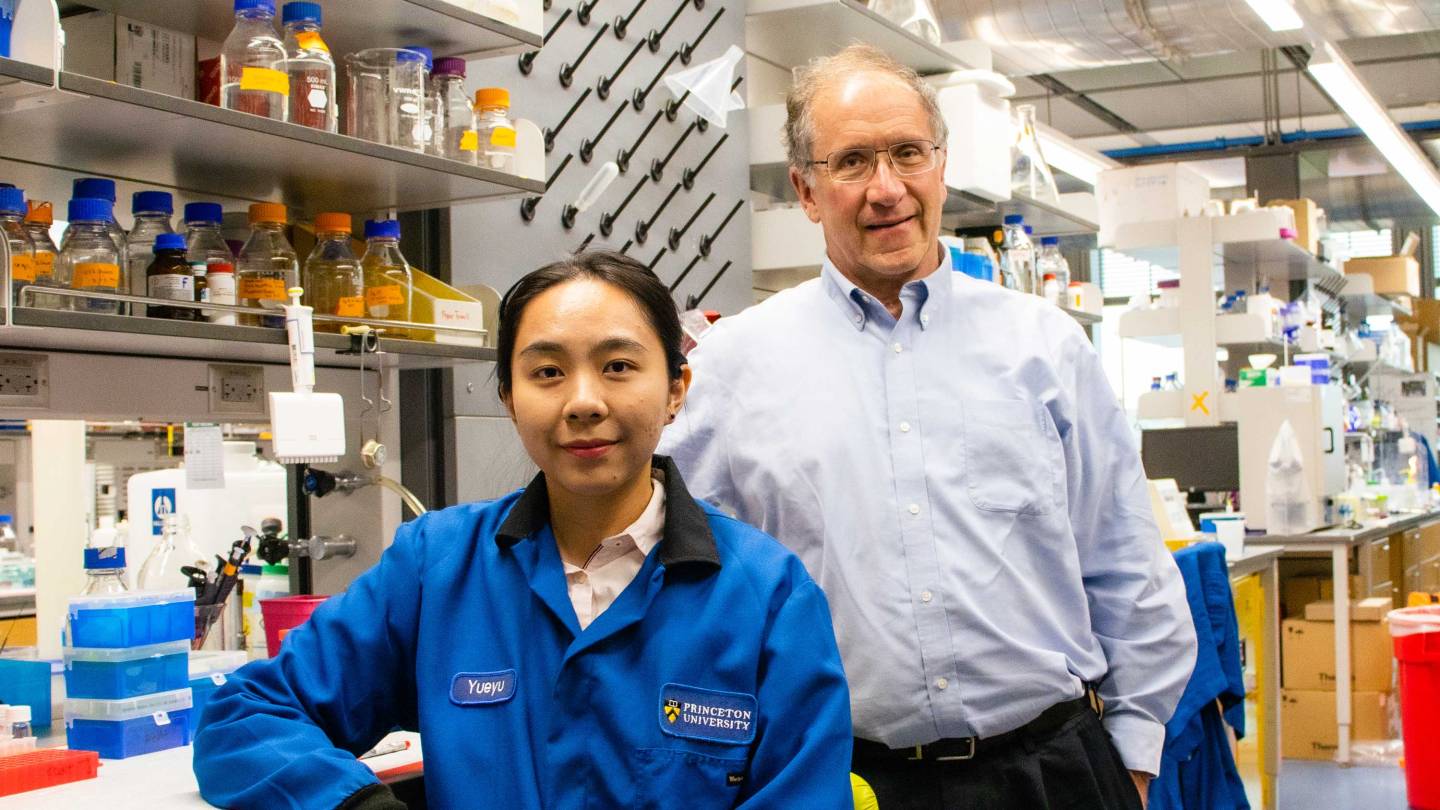The photograph captures a detailed glimpse into a scientific laboratory. In the forefront, a young Asian woman with her hair pulled back is seated at a lab bench, donning a blue lab coat that features a name tag and a Princeton University insignia. Standing behind her is an older man, likely the principal investigator given his age; he sports glasses and a light blue Oxford long-sleeve shirt paired with dark slacks. The man appears to be bald or balding. Both individuals are looking directly at the camera. Surrounding them is a meticulously organized lab, complete with various science equipment such as beakers, vials, test tubes, and drying racks with funnels and tubes. The backdrop includes fluorescent lighting, numerous workbenches, and shelves filled with bottles and scientific supplies, all contributing to the sterile and clean environment of the laboratory.